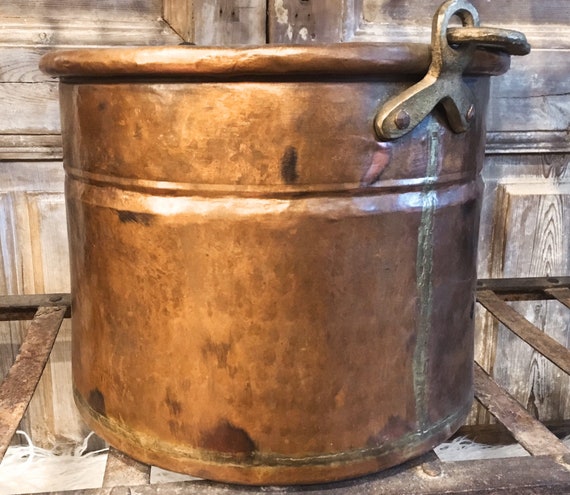The image features what seems to be a wide, metallic copper bucket with a rounded rim and visible rivets where the handle attaches. The handle itself looks slightly rusted, and the bucket displays an uneven sheen with darker spots and a vertical brown mark running down its side. It appears to have had some aging effects applied to give it a more rustic appearance, although it is likely a reproduction rather than an antique piece. The bucket, which may also be considered a cooking pot, is placed on an old metal wire bed frame, set against a rustic wooden wall that appears to be part of an old structure or possibly staged as cabinet doors. There is a visible chain structure on the right side of the bucket, suggesting functionality for attaching to a rope or other apparatus. This setup strongly suggests that the image is designed as a product photo, likely for an online marketplace such as Etsy.